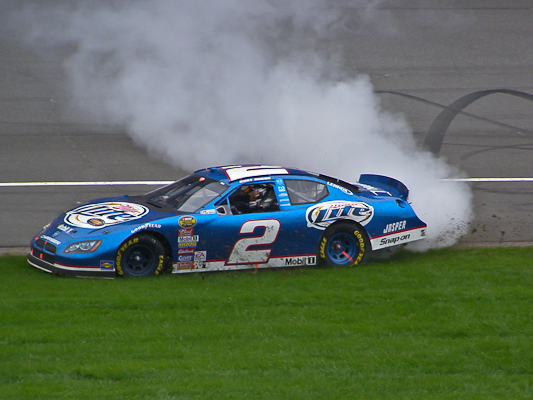This image captures a dramatic moment involving a shiny blue NASCAR race car, characterized by its prominent white number '2' displayed on both the roof and driver's side door. The car, primarily shown from the driver's side, features a large Miller Lite logo in a white circle on its front hood, with additional 'Miller Lite' branding above the rear tire. Other sponsor logos such as Jasper Snap-on and Mobil are visibly positioned around the rear and front tires.

The race car is centrally placed in the image, situated partially on a grassy area adjacent to an asphalt racetrack. Distinct skid marks trace the car's path from the track onto the grass, indicating an accident. A substantial plume of white and grey smoke billows from the tailpipe, enveloping the scene and suggesting the car is experiencing mechanical trouble. The car's driver, visible inside and wearing a helmet, adds a human element to the scene. The image is set outdoors in the daytime, with the vivid colors of green grass, grey asphalt, and the colorful sponsor logos adding contrast and detail to the dramatic situation.